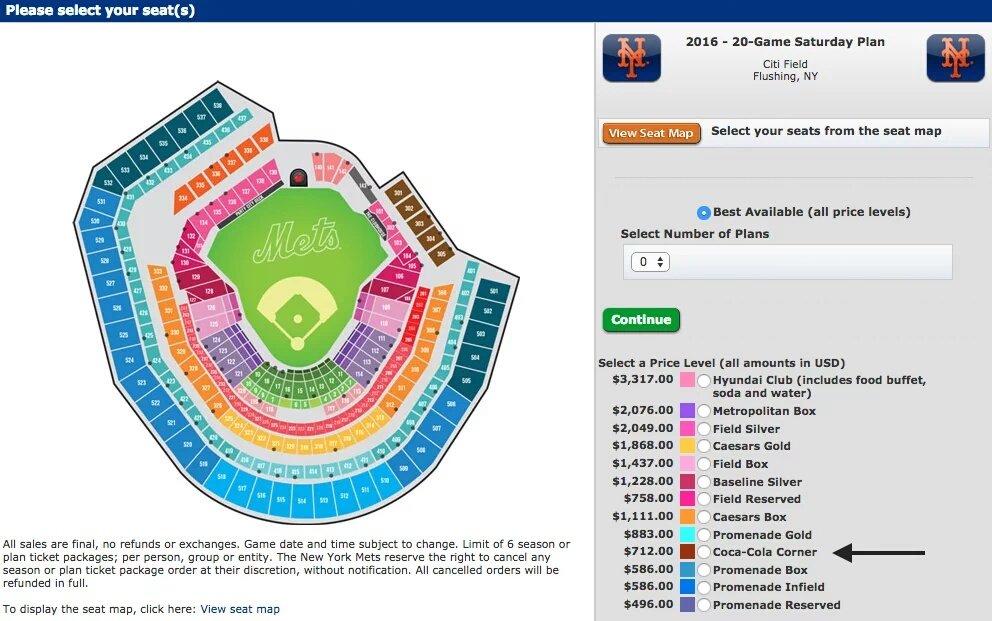This screenshot captures the ticket purchasing webpage for the New York Mets. It prominently features a detailed baseball stadium map of Citi Field in Flushing, New York, with sections highlighted in various colors such as pink, purple, yellow, teal, and blue, each representing different pricing codes. The color-coded map offers a visual guide to seat pricing for a 2016 "Saturday Plan," covering 20 games. Ticket prices range from $3,317 to $496.

Below the stadium map, important information is indicated: all sales are final with no refunds or exchanges permitted. Game dates and times are subject to change. Furthermore, there's a restriction of up to six season or plan ticket packages per individual, group, or entity. The New York Mets also reserve the right to cancel any order for season or plan tickets at their discretion, with full refunds provided for canceled orders. 

To explore the seating map in more detail, users are invited to click on a link labeled "View Seat Map."